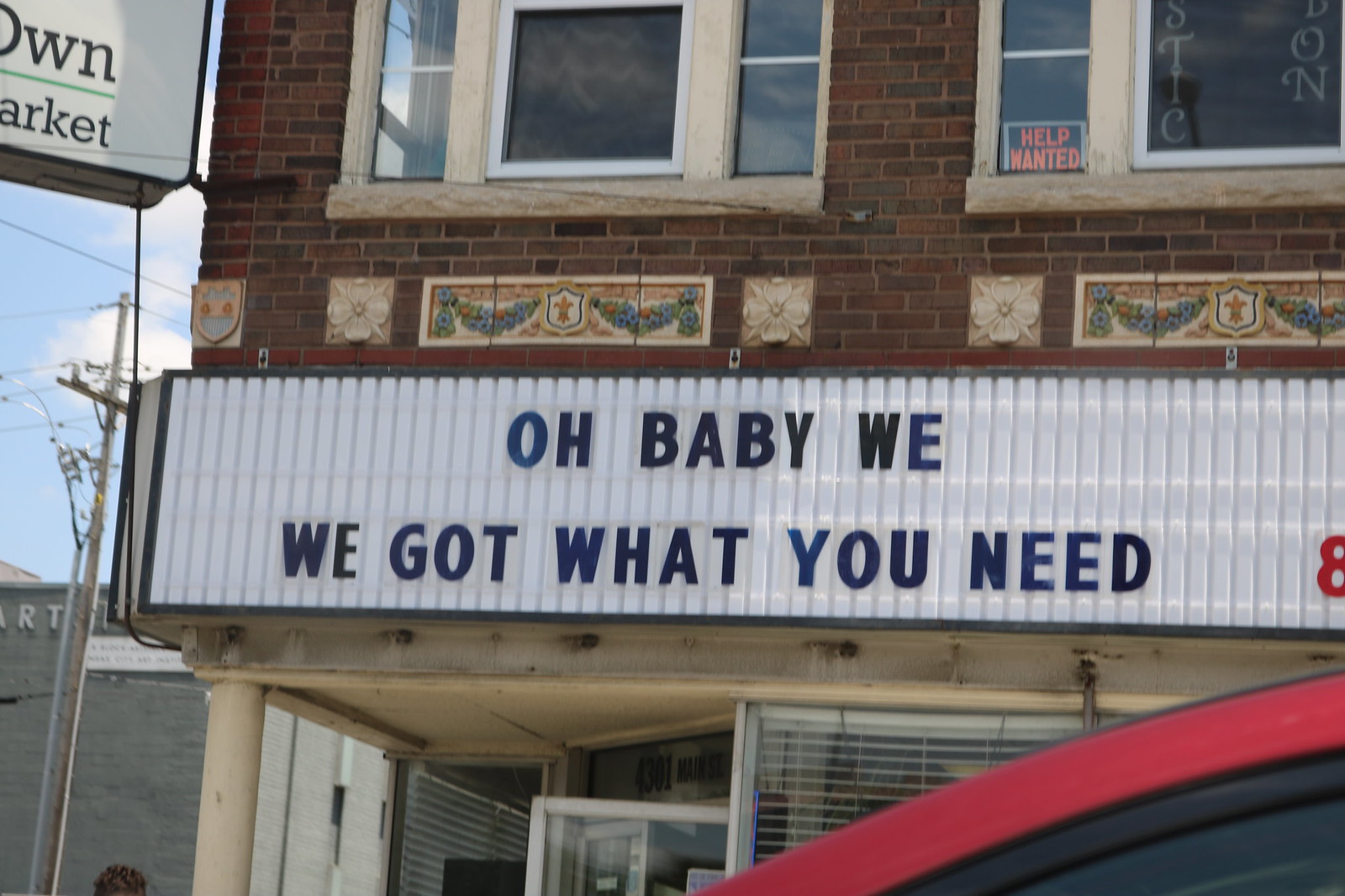In this photograph, we see a charming yet slightly run-down storefront on the corner of a decorative brick building. The primary sign, hanging to the left and adorned with a mix of black and blue text, reads, "Owen OWN Market." Above the entrance door, propped open invitingly at the corner, another large sign enthusiastically declares, "Oh baby, we got what you need," with a notable red number eight adjacent to the text. Additionally, a smaller sign upstairs indicates a "Help Wanted" notice. The building, though aged, features ornate brickwork with floral patterns and various symbols, hinting at its storied past. The combination of the intricate details of the brickwork and the nostalgic feel of the market's signs creates a snapshot of a quintessential old neighborhood gem.